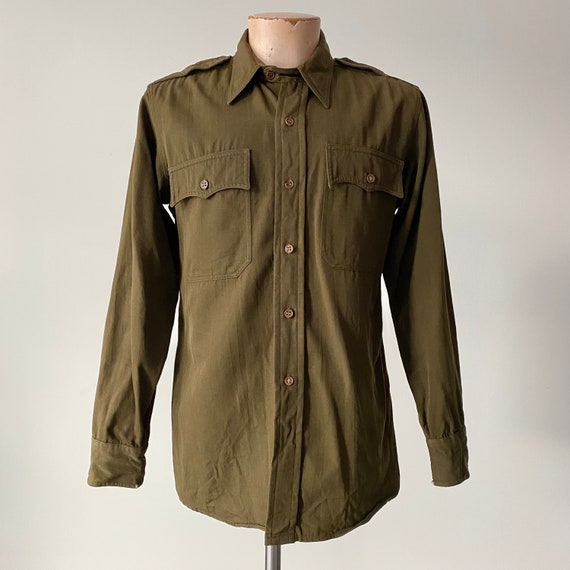This image features a mannequin displaying a long-sleeved, collared shirt in a distinctive brownish-green hue, reminiscent of army green. The shirt, which exudes a utilitarian style, includes functional details such as buttoned flaps on the shoulders and buttoned pockets on each side of the chest. It fastens down the front with six evenly spaced buttons, aligning with its classic yet rugged aesthetic. Both sleeve cuffs are buttoned, eschewing cuff links for a more casual finish. The mannequin itself has a wooden flat-top head, a skin-toned neck, and is supported by a sleek, silver metal bar, all set against a pristine white background.